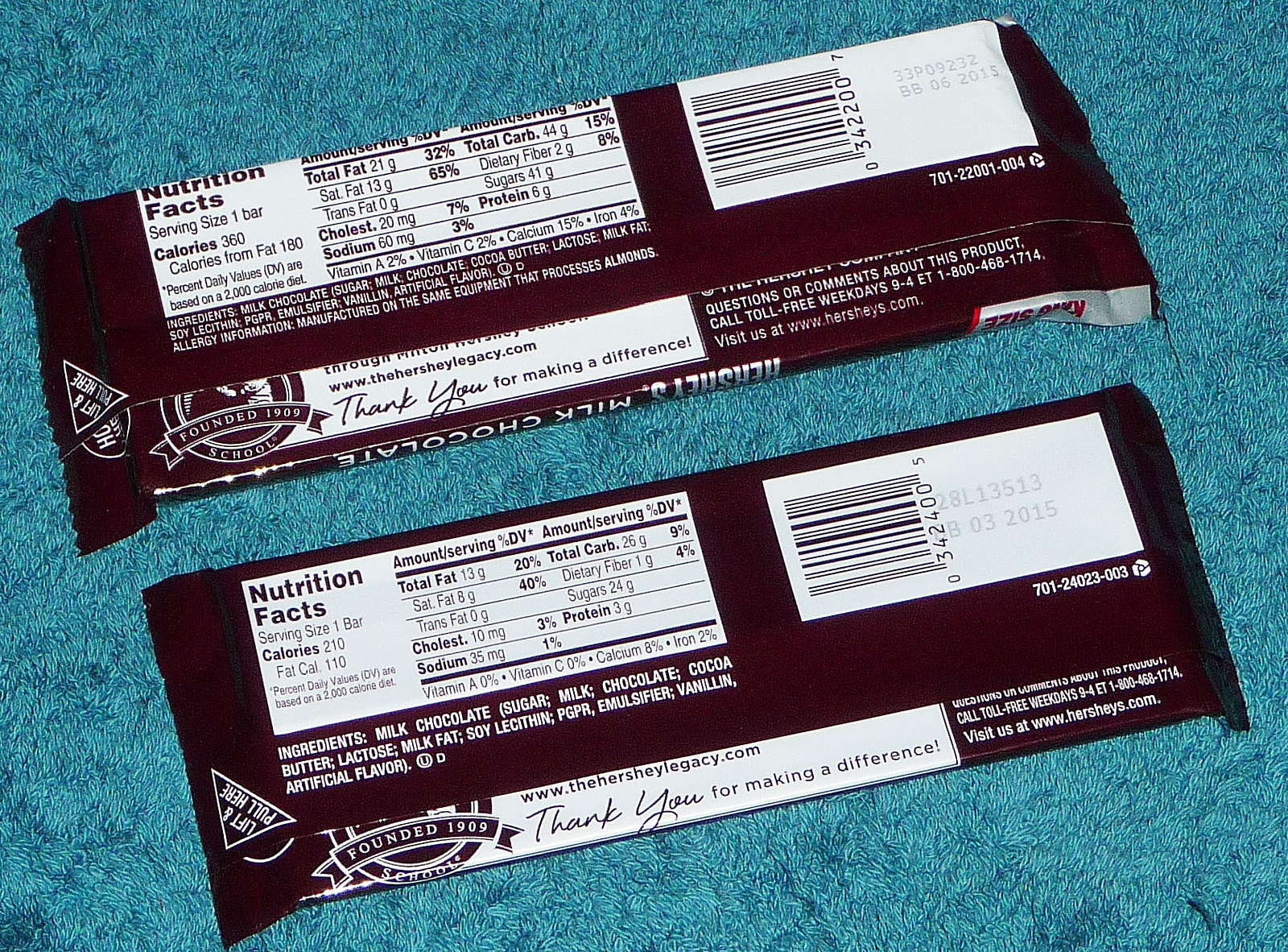The image features a vibrant blue background with two Hershey bars positioned diagonally across it. The bars are flipped to reveal the reverse side of their packaging. The wrappers are the iconic black with white labeling. In the upper left corner of each wrapper, a white panel displays the Nutrition Facts. The upper right corner features a UPC barcode. In the bottom right corner, there is a designated area containing a phone number for consumer comments or questions. The lower left corner is adorned with a circular medallion, stating "Founded in 1989" with the word “school” below it. The Hershey bar at the top is noticeably thicker than the one at the bottom, which appears to be a smaller-sized candy bar.